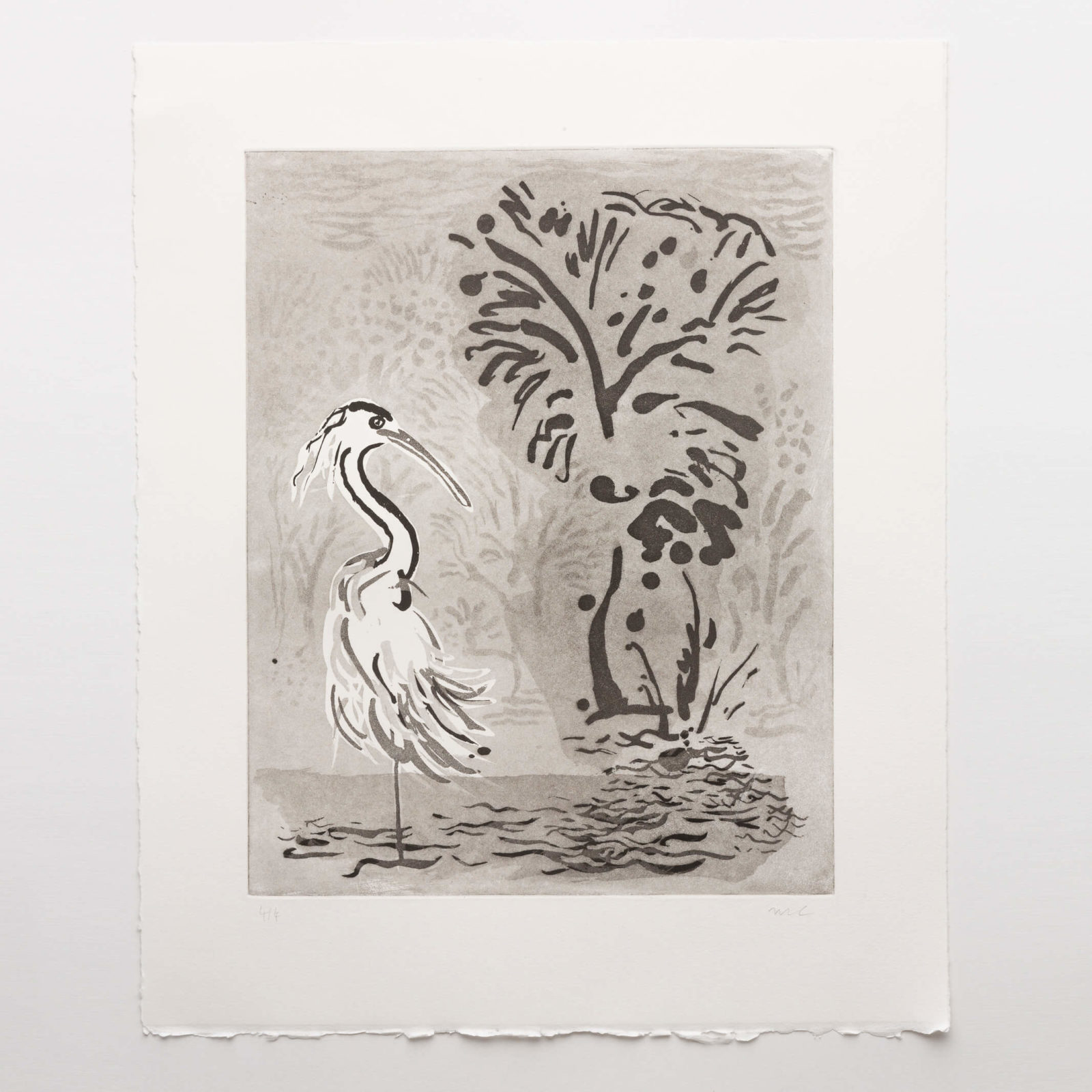This artwork, perhaps rendered in pen and ink or watercolor, is displayed on a white table or affixed to a white wall. The rectangular piece of paper is neatly torn at the bottom and cleanly cut on the other sides. The monochromatic image depicts a stylized bird, likely an egret or ibis, characterized by its large, narrow bill and elegant, elongated neck. The bird is facing to the right and is standing upright on one leg in a small pool of water. Its feathers are depicted with a flowing, billowy effect. To the right of the bird, there is a vaguely defined, perhaps abstract tree-like shape with a trunk and branching marks that suggest foliage. The image presents a combination of detailed and abstract elements, with the bird being the most realistic feature amidst the abstract representations of water, sky, and vegetation.